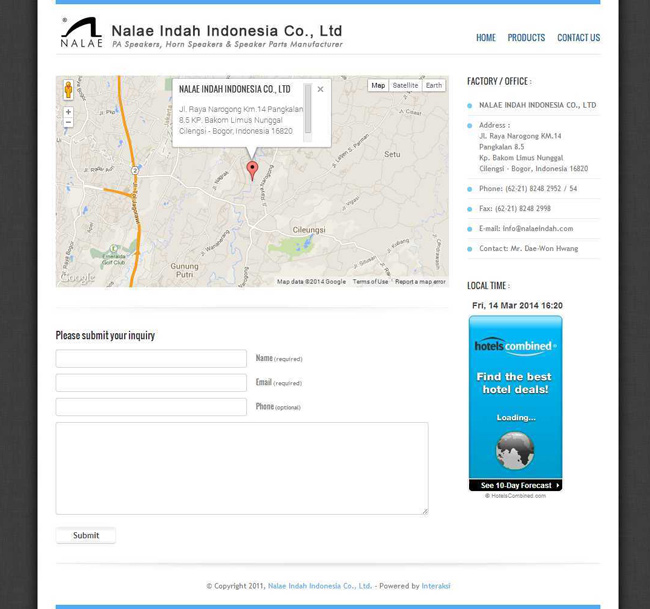The image portrays the homepage of the Nali Indiha Indonesia Co., LTD website. At the top, there is a detailed map with a prominent pin marking the location of Nali Indian Modesta County LTD, centrally positioned. The map also features various annotated areas on the side, with yellow lines tracing different roadways to illustrate routes to the location. Below the map, the company's address is displayed.

Toward the bottom of the webpage, there is an inquiry submission section. This section includes input fields for a name, email, and photo, along with a large text area for typing a detailed message. The submission process is finalized by clicking the 'Submit' button.

Additionally, an advertisement for Hotels Combined is featured at the very bottom, encouraging users to "find the best hotel deals." This ad displays a loading symbol and an image of the Earth against a striking royal blue background. Above the map, an image highlights the factory office area, giving a clearer visual representation of the company's facilities.